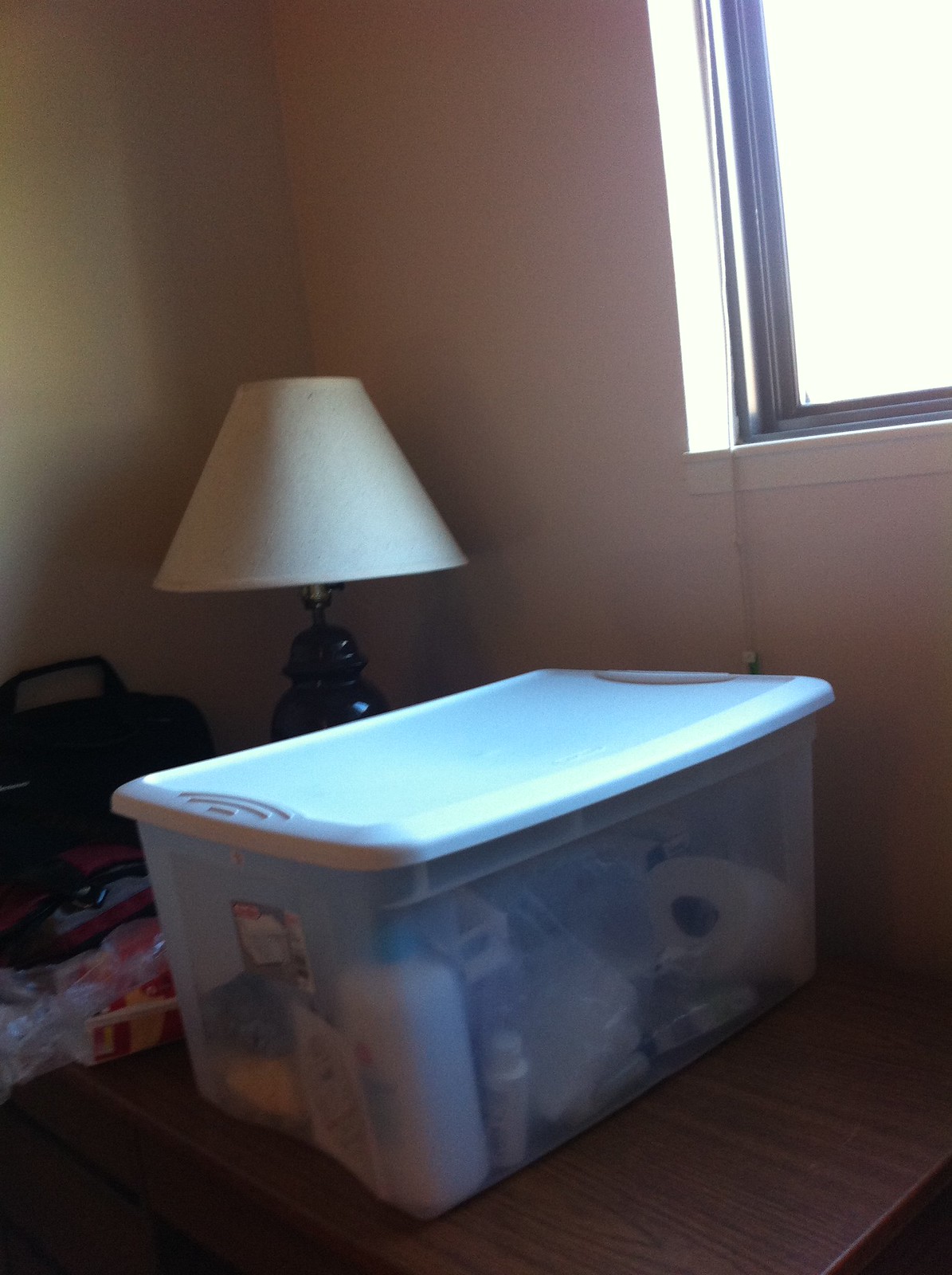In the back of the picture, a sleek black lamp with a white shade stands elegantly. Dominating the foreground, a dark wooden coffee table hosts a variety of items. Atop the table, a large plastic storage tub with a lid contains an assortment of cleaning and first aid supplies. Adjacent to the tub sits a clear plastic bag featuring a conspicuous sticker, and further down, a sizable duffel bag with a convenient handle is placed. The walls of the room are painted a crisp white, providing a bright and clean backdrop. Centrally above the coffee table and storage tub, a slider window with a brown metal frame is positioned, designed to open side-to-side rather than up and down. A dangling string for the window shade can be seen at the bottom of the window, completing the tidy and organized scene.